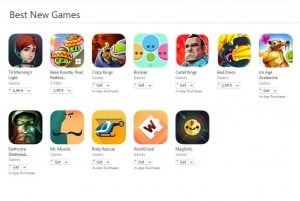The image features a header titled "Best New Games" with an underline accentuating the text. Below the header, there are two rows showcasing different game titles, with the top row containing seven thumbnails and the bottom row containing five. Each game is represented by a thumbnail image with its title displayed underneath, though the overall image quality is highly blurred, making the specific game titles indiscernible.

In the top left thumbnail, there's an image of a person with short red hair. To the immediate right, the next thumbnail displays small green faces that appear to be wearing sombreros. The following thumbnail on the row is unclear. The subsequent image, set against a blue background, features an orange, blue, and purple circle with eyes, seemingly observing a green circle. Lastly, the far-right thumbnail of the top row shows a heavyset man with a gray mustache, wearing a blue shirt against a red background.